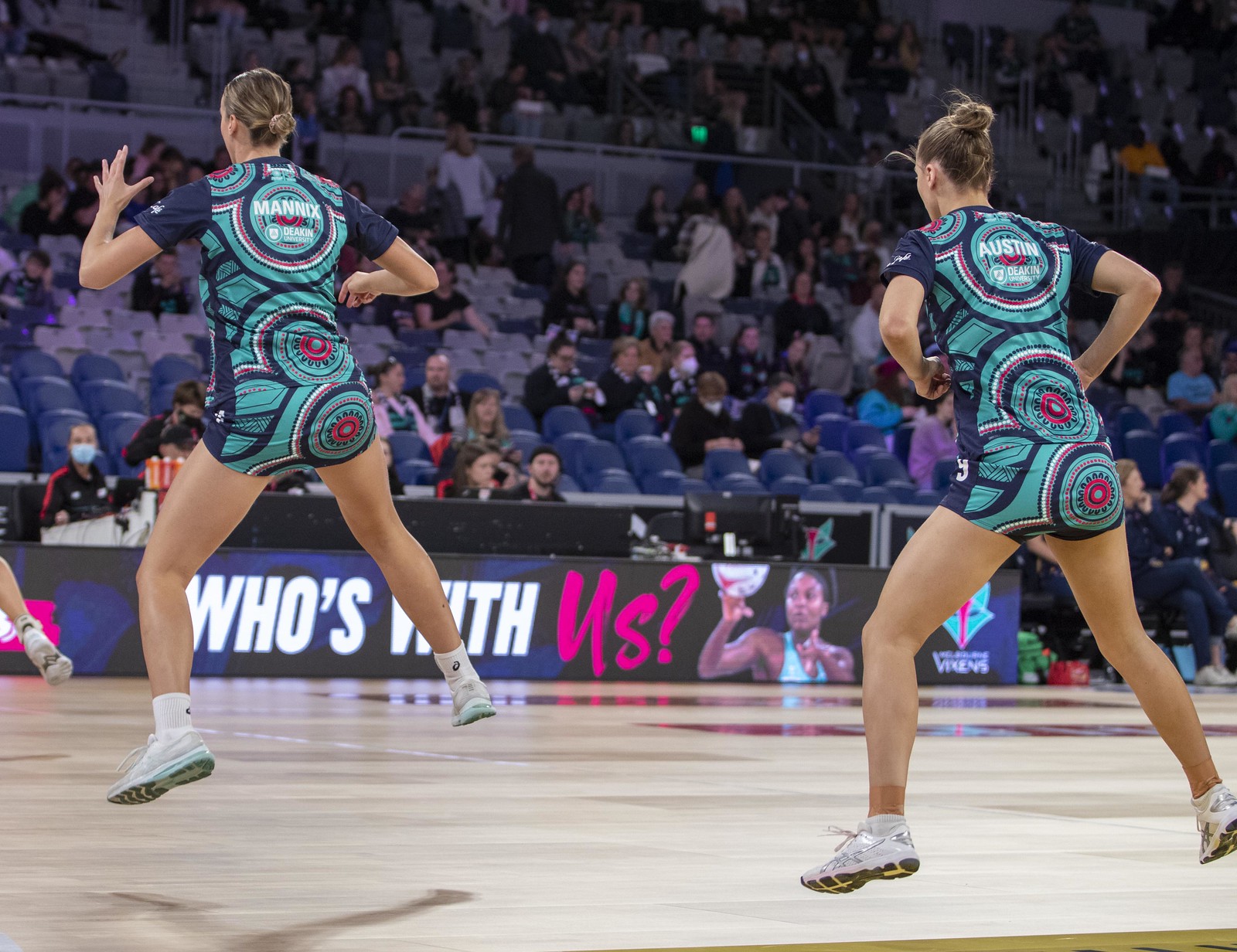The photograph captures an intense moment of an indoor basketball game, featuring two girls in the foreground with their backs to the camera, each mid-jump. The players are wearing vibrant, matching uniforms adorned with shades of blue, dark blue, white, and noticeable pink accents. The left player's jersey reads "Mannix" in white text, while the right player's jersey reads "Austin." They are performing on a light brown wooden court, adding a warm contrast to their colorful attire. Above them, a prominent banner displays an image of a woman and the phrase, "Who's with us?" with "us" highlighted in pink. A half-filled audience can be seen seated in blue and purple chairs, intently watching the game unfold.